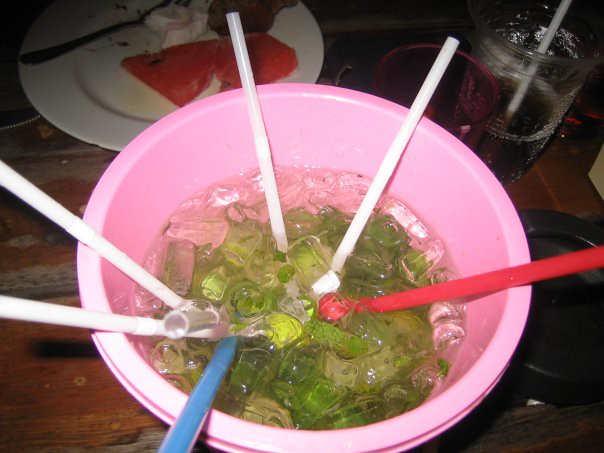In the center of the photograph is a large pink bowl on a brown wooden table, filled with small cylindrical ice cubes and a dark green, unidentifiable substance underneath, which is slightly obscured by the ice. Seven straws extend from the bowl, likely indicating a shared dragon bowl drink: five straws are white, one is blue, and one is red. Behind the bowl is a white plate with what appears to be leftover food, possibly tomato slices or something red, white, and dark, with a fork or spoon laying across it. To the right of the bowl, there is a glass filled with a dark liquid and a white straw, and partially obscured behind the bowl is another pink glass with an indistinguishable amount of liquid. The setting suggests it's post-meal, given the plate and the additional drink glasses with condensation and bubbles.